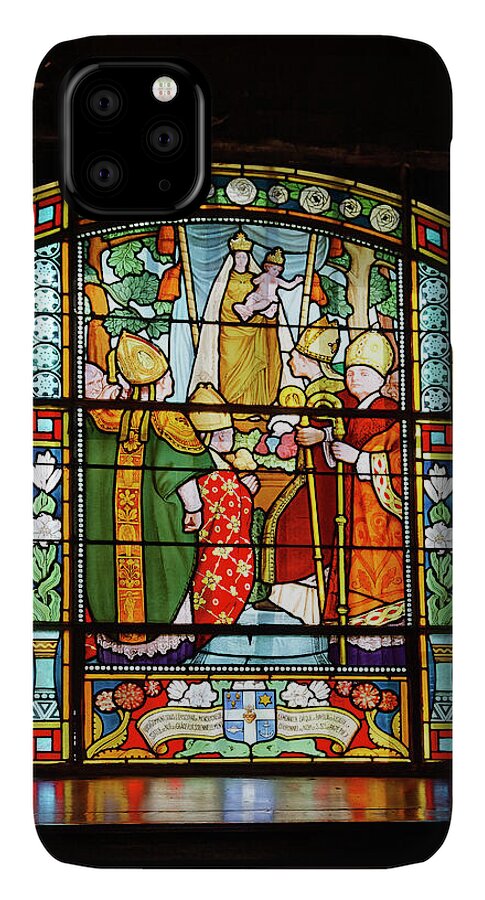This is a black cell phone cover featuring a vibrant depiction of a stained glass window with intricate divisions marked by black lines mimicking the lead supports of a real window. The centerpiece of the stained glass imagery depicts a religious scene dominated by the figures of a crowned woman, likely Mary, with a long white veil, holding a baby with a golden crown, presumably Jesus. Standing in front of her are four men, possibly disciples or religious figures. On the far left is a man in a green gown adorned with gold and red decorations wearing a tall, pointed, priest-like cap. Next to him kneels a man clad in a red cape embellished with gold flowers, also wearing a high pointed gold cap. The third man, slightly bent, is dressed in a red gown and holds a golden staff, capped with a similar gold hat. The fourth man on the right wears a red cape with white bands, also holding a staff and donning a high golden hat. The stained glass design features an array of rich colors—greens, reds, golds, blues, and whites—creating a vivid, multi-colored display. At the lower part of the scene, there appears to be a blue emblem surrounded by primary colored decorations, possibly flowers, along with an unreadable banner. The background includes painted leaves, further adding to the detailed craftsmanship of this religious artwork.